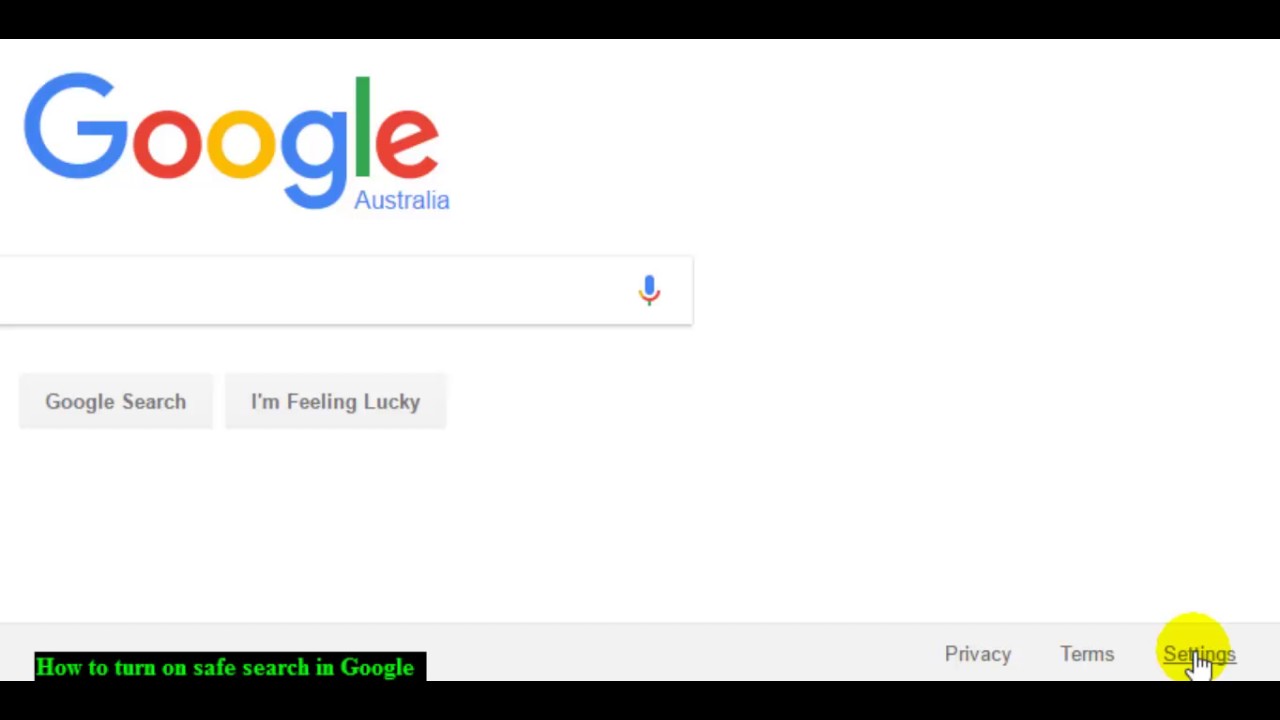The image is a screencap of the Google homepage, distinctively marked by the iconic Google logo positioned at the top-left corner. The logo features the multi-colored letters: a blue 'G', a red 'O', a yellow 'O', another blue 'G', a green 'L', and a red 'E'. Just below, the word "Australia" is written in blue, indicating the regional variant of the search engine.

Central to the image is the familiar rectangular search bar, stretching from the very left to the center. The search bar is entirely empty, blending seamlessly into the white background. At the far right edge of the search bar is a gray microphone icon, signifying the option for voice search.

Beneath the search bar, two gray-text buttons appear: "Google Search" on the left and "I'm Feeling Lucky" on the right. Down at the very bottom left of the screen, there is a black bar containing green text that reads "How to turn on SafeSearch in Google". 

To the right of this text, various links are listed in white: "Privacy," "Terms," and "Settings." The "Settings" link is notably enclosed in a yellow circle, indicating it is currently highlighted, with the cursor positioned over it. The entire screencap is bordered by a black frame at both the top and bottom edges, providing a clear boundary for the image.